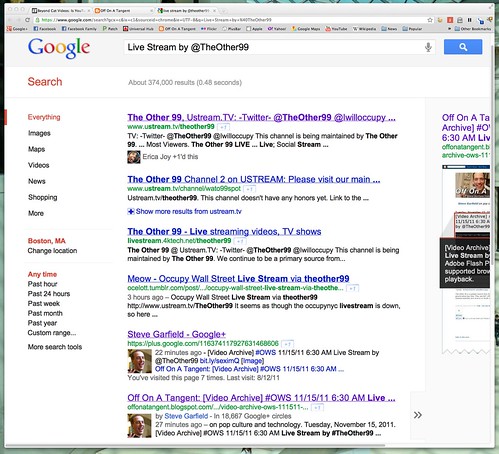This image is a detailed screenshot of a Google search results page. At the top of the browser, three tabs are visible. The search is conducted on Google, with the iconic Google logo prominently displayed. The search query entered in the bar reads "live stream by at the other 99," yielding approximately 374,000 results.

On the left side, the sidebar features various search filters and tools including options for "Everything," "Images," "Maps," "Videos," "News," "Shopping," and others. The user can also change the location setting, which is presently set to "Boston, MA," and refine the search by time frames such as "Anytime," "Past hour," "Past 24 hours," "Past week," "Past month," "Past year," and "Custom range."

The listed search results illustrate different links related to "the other 99" live streams and online presence:
1. A visited link to "The Other 99 on UstreamTV" noted in purple.
2. An unvisited link directing to "The Other 99, Channel 2 on Ustream."
3. Another unvisited link titled "The Other 99: Live streaming videos, TV shows."
4. An unvisited link for "Occupy Wall Street Live Stream via The Other 99."
5. A visited "Steve Garfield Google+" link, also marked in purple.
6. A visited link to "Off on a Tangent" featuring a video archive tagged with "#OWS 11/15/11 6:30 AM live," also displayed in purple.

This comprehensive snapshot captures the essence of a search centered on live streaming content provided by "The Other 99," reflecting the user’s past interactions with some of the displayed links.